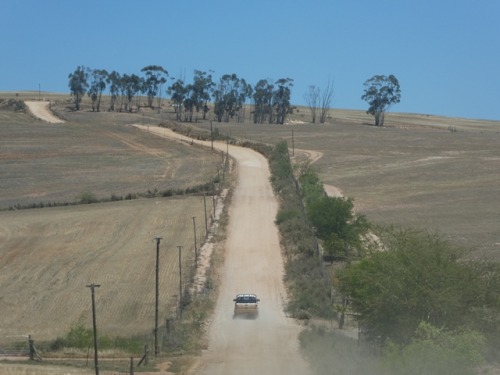In this square aerial image, a wide, even dirt road, potentially at the top of a low hill, stretches upward from the bottom center and curves to the upper left. A SUV, likely gold or silver, travels in the middle, kicking up dust along the way. Flanking the road are brown fields, surrounded by green-leaved bushes and sparse trees on the right. On the opposite side, utility poles with lights line the road, hinting at nearby settlement. The background features additional trees and tall, thin trees, possibly eucalyptus, under a clear, solid blue sky devoid of clouds. No animals or buildings interrupt the serene, semi-settled landscape.